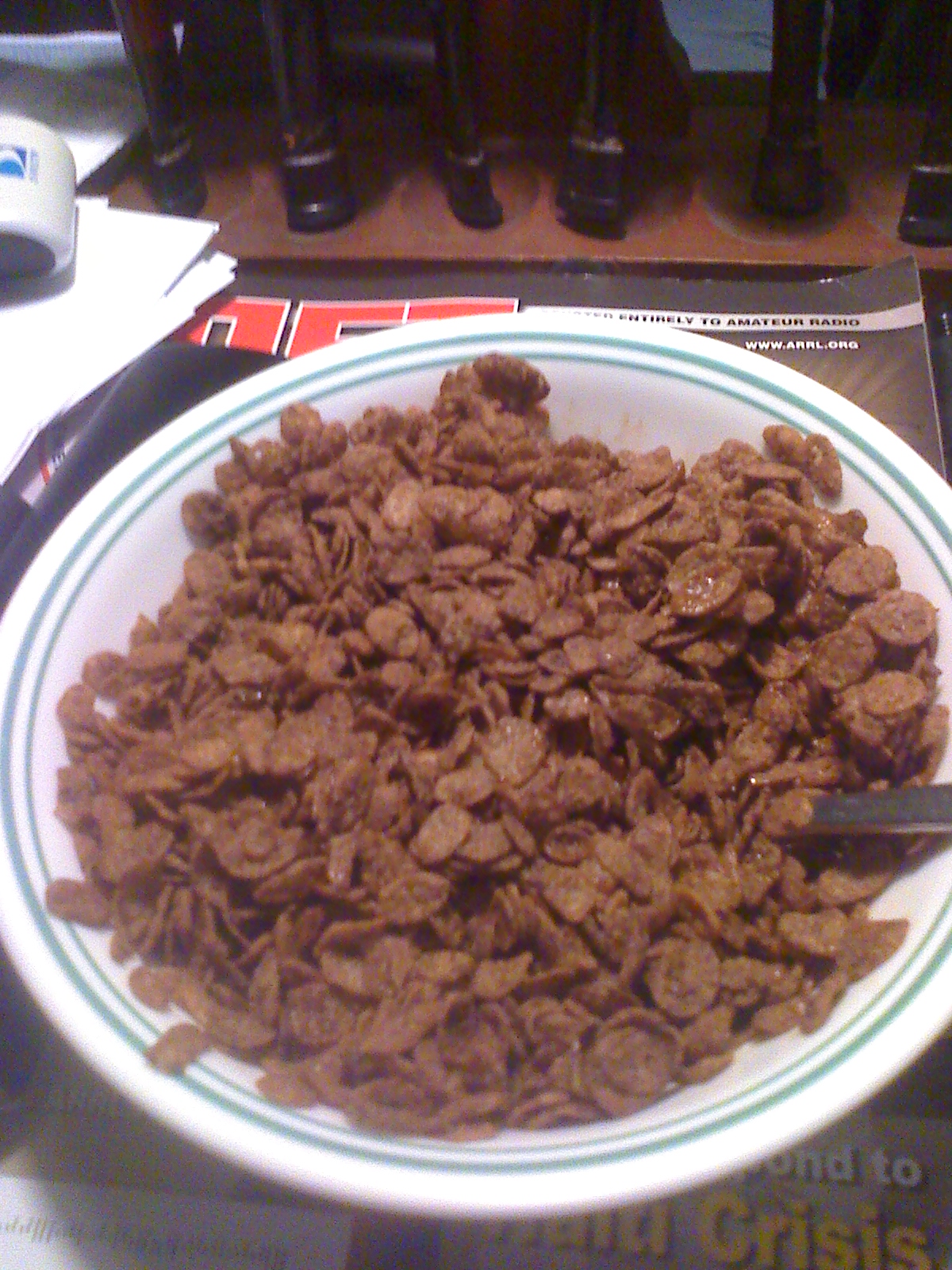In the image, there is a white ceramic bowl with two circular light green borders, containing what appears to be Cocoa Pebbles cereal. The bowl, which is large and shallow, is partly obscuring a magazine. The magazine prominently features a headline about the Haiti crisis and includes the text "Amateur Radio www.arrl.org." Surrounding the bowl on the cluttered desk are various scattered items, including what looks like a roll of stamps and some papers. In the upper left corner of the image, a partially visible DirecTV logo is seen on a white surface. The background features a wooden structure with vertical support beams, resembling the back of a chair or a railing, which is dark brown and slightly blurred.